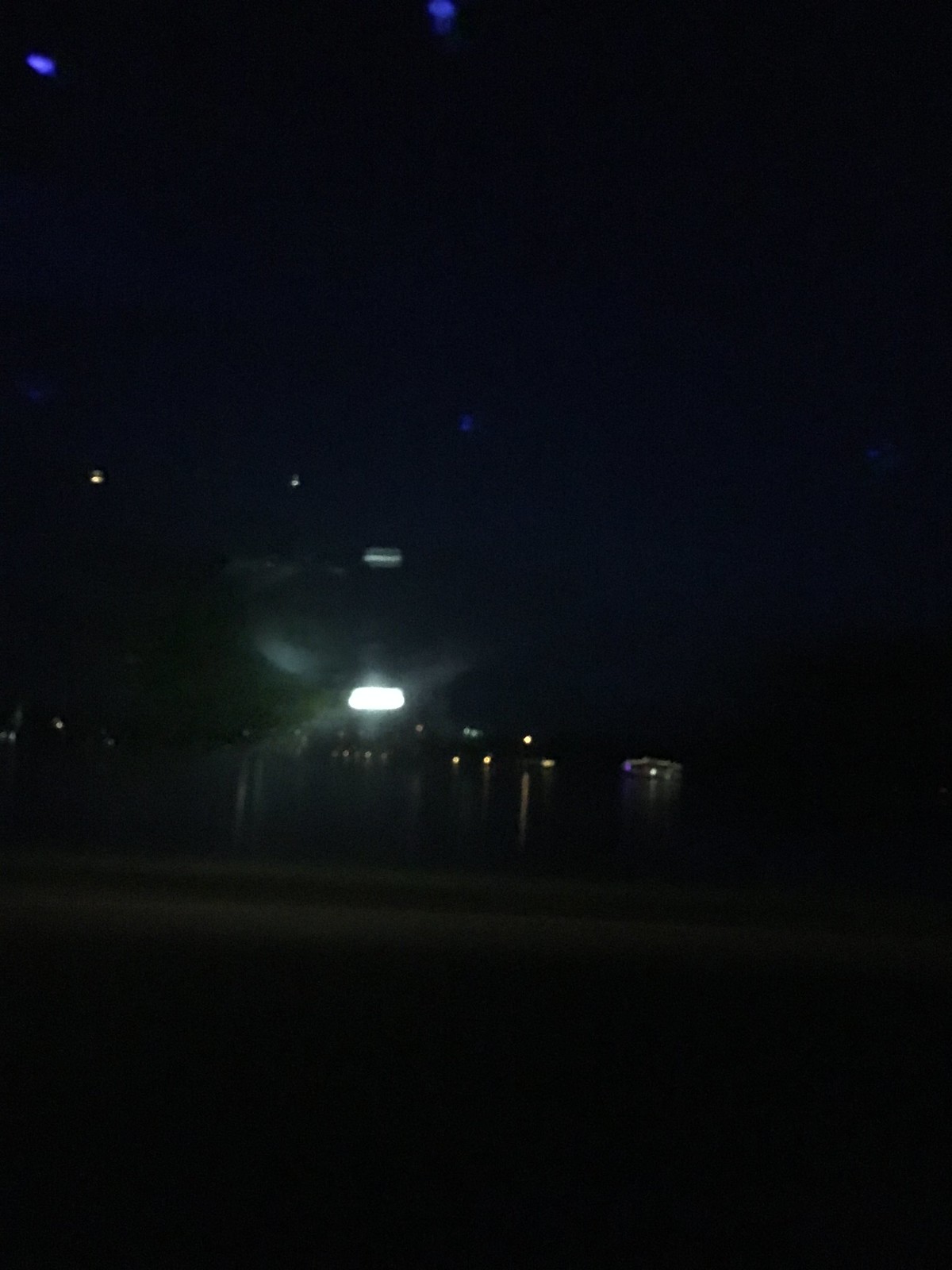This image, presented in portrait orientation, captures a nighttime scene from one side of a street overlooking a body of water, likely a still lake or river. The photograph is quite blurry and appears to have been taken through glass, contributing to the reflections visible in the frame. Across the street and perhaps a sidewalk, the image reveals several lights dotting the distant shore, with some of them casting shimmering reflections on the water's surface.

In the center of the composition, a significantly brighter rectangular light dominates the scene, emitting streaky rays that pierce through the darkness. Besides this central light, there are other smaller lights visible, including a couple of blue ones at the top edge of the frame and possibly a light on a boat on the water. Despite the overall darkness cloaking the photograph, the reflections and sporadic lights provide a glimpse into the nighttime environment surrounding the serene body of water.